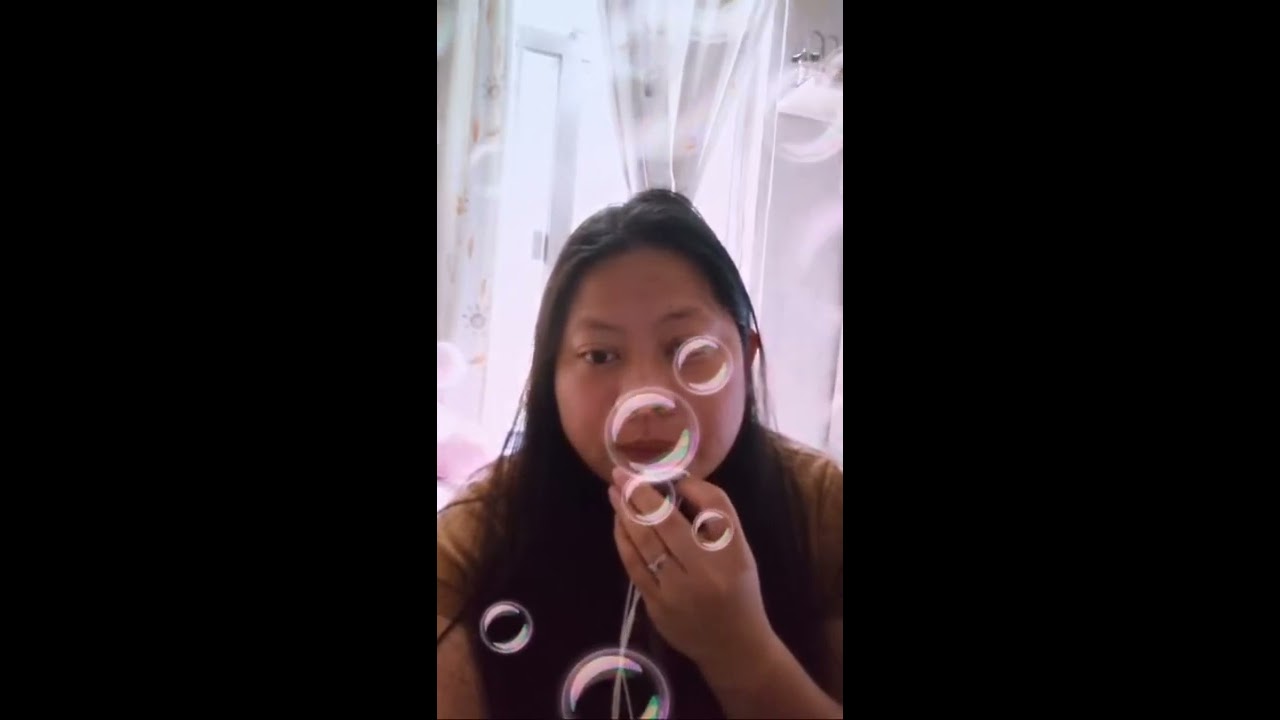The image is a still from a portrait mode video featuring a girl with a roundish face and long black hair cascading down past her chest. The left and right thirds of the image are taken up by large black empty spaces, making a black rectangular border around the central segment of the photo. In the middle third, the girl is seated in a room in front of a window through which sunlight is streaming. The window has white curtains with some sort of pattern, partially visible and slightly blurry. The girl is wearing a beige t-shirt and has a ring on her left hand. Her left hand is bent up, touching her face, and she appears to be interacting with a bubble filter effect, as there are bubbles directly in front of her face, slightly above and below her, and on her hair and shirt. A white wire, possibly from earphones, dangles from her hand.